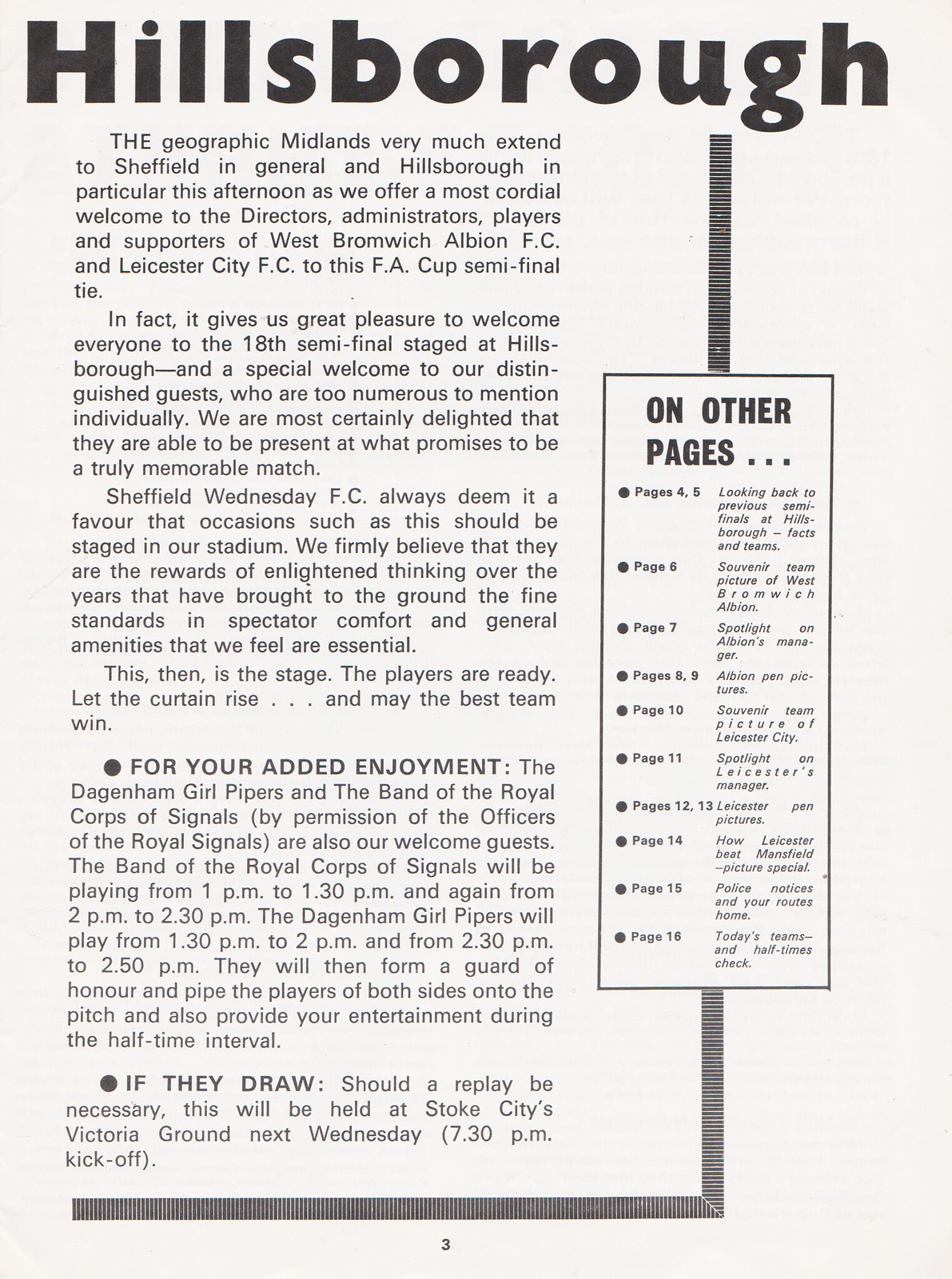This scanned image is from an old game day program or magazine, specifically page three. Dominating the top of the page, in large, bold text, is the word "Hillsborough." The article beneath this heading consists of multiple paragraphs and begins with the sentence, "The geographic Midlands very much extend to Sheffield in general and Hillsborough in particular this afternoon, as we offer a most cordial welcome to the directors, administrators, players and supporters of West Bromwich Albion FC and Leicester City FC to this FA Cup semifinal tie." The right side of the page features a vertically aligned rectangular section bordered in black with the heading "On Other Pages." This index lists the contents of other pages, including highlights such as a look back at previous semifinals at Hillsborough on pages 4-5, a souvenir team picture of West Bromwich Albion on page 6, and similarly detailed descriptions leading up to page 16. Bullet points on the left side provide additional navigation details. The bottom of the page is marked with the number three.